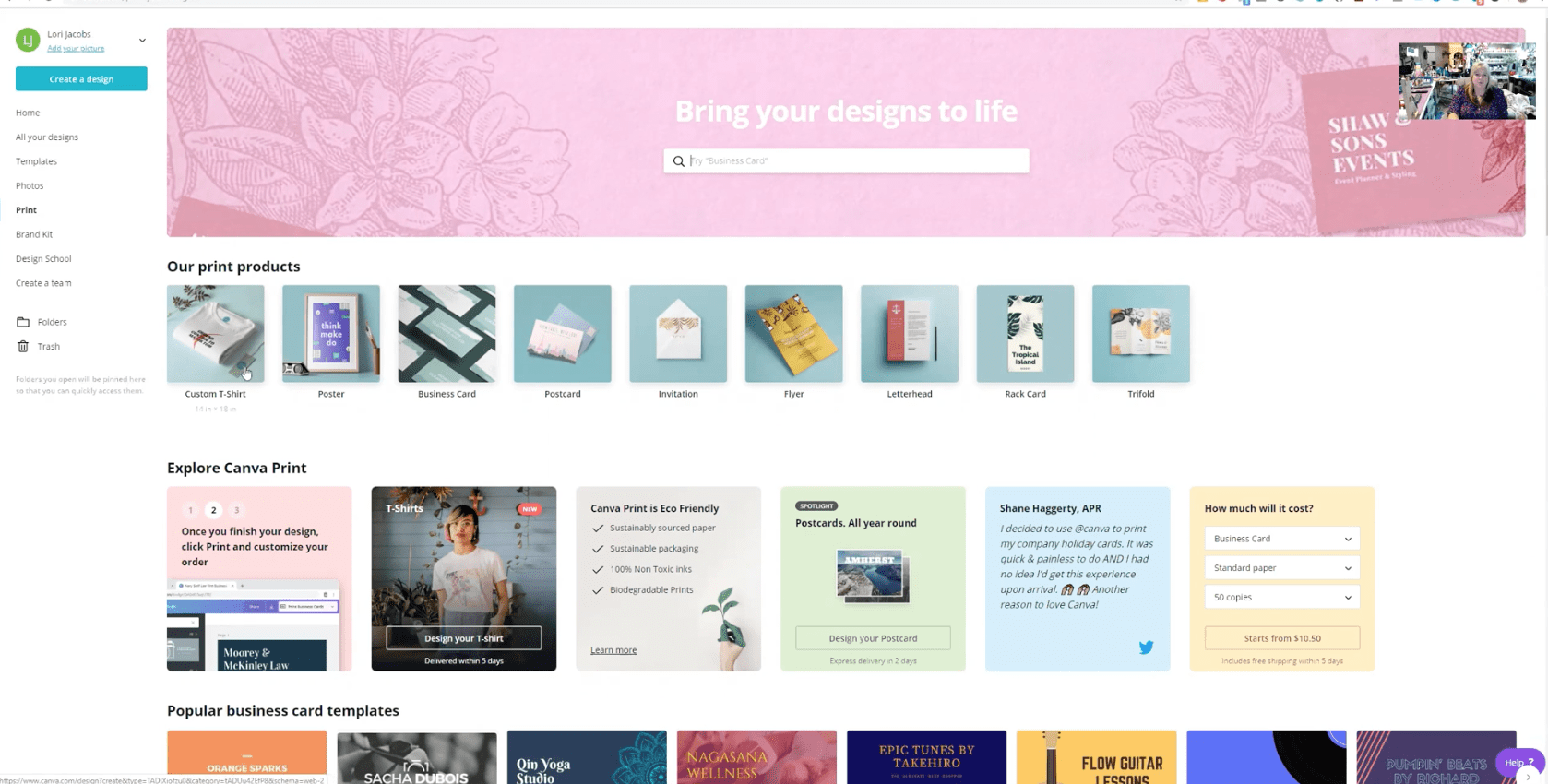This screenshot captures a section of the Canva website showcasing its various print services. The site allows users to print photos, journals, and home decorations, although the specific web address or brand name is not made visible initially. The page prominently features a heading, "Our Print Products," under which an array of print options are listed, including envelopes, cards, brochures, flyers, invitations, postcards, and custom t-shirts.

Further down the page, the brand identity is revealed through a statement, "Explore Canva Print," highlighting Canva's eco-friendly print services, such as year-round postcard printing. This section includes a testimonial from an individual named Shane Haggerty, though the text is notably small and hard to read.

Additionally, the page offers a cost estimation tool where users can select from various options, like business cards on standard paper, to ascertain the price of their desired print project through a drop-down menu. On the right-hand side, the website encourages users to create an account for accessing specific features, which might include managing photo folders, checking project statuses, and reviewing discarded items, despite the text being minuscule and challenging to decipher.